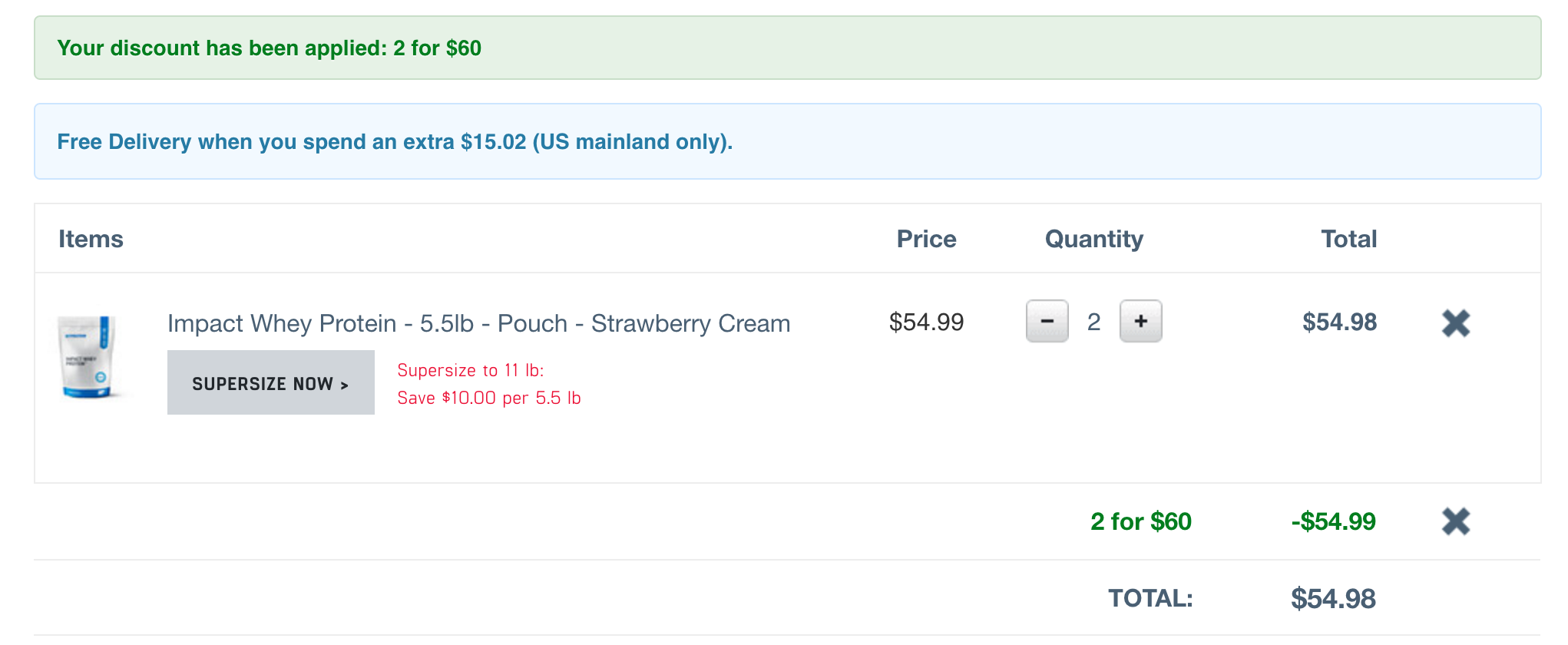The screenshot showcases a shopping cart summary on a website with a white background. At the top, a gray rectangle highlights the message "Your discount has been applied." Below this, it states an offer: "Two for $60." A blue rectangle next indicates, "Free delivery when you spend an extra $15.02 (U.S. mainland only)."

The items listed include "Impact Whey Protein, Whey, 5.5 LB pouch, Strawberry Cream" with an option labeled "Supersized Now" in a gray rectangle. This option allows for upgrading to "11 LB" and offers a savings of "$10 per 5.5 LB." The current price for the 5.5 LB pouch is marked as "$54.99."

Two units of the whey protein are in the cart. Each unit's quantity can be adjusted with a negative sign on the left and a plus sign on the right. The current subtotal is "$54.98," bundled with a green note: "Two for $60." Below the total, there’s a discount showing "-$54.99," leading to a final total of "$54.98."